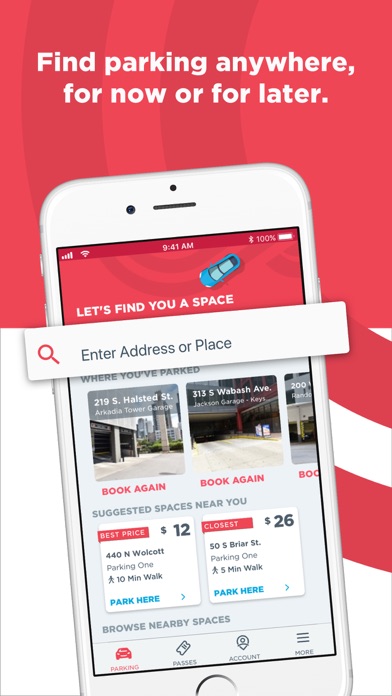**Detailed Caption:**

The image portrays a vertical advertisement, designed to catch the eye of someone casually scrolling through a feed. The background features a striking red hue, enhancing the visibility of the main elements. Central to the image is a white smartphone prominently displayed. The screen of the smartphone shows a parking app interface. 

At the top of the smartphone screen, a white search bar with a red magnifying glass icon and gray text that reads "Enter address or place" is visible. The search bar extends off the edge of the smartphone, emphasizing its importance.

Directly beneath this search bar, bold white text on a red background encourages action with the phrase, "Let's find you a space." Displayed below this message is an image of a blue sedan, representing a parked car.

Further down, the screen shares a list of recently parked locations with the options to "Book Again." The locations listed are:
1. 20 to 19 South Halsted Street, Arcadia Tower Garage - "Book Again"
2. 313 South Wabash Avenue, Jackson Garage - "Book Again"
A third option is partially obscured, trailing off the visible screen.

At the bottom, suggested parking spaces nearby are highlighted:
- **Best Price**: $12, 440 North Wolcott Parking, 10-minute walk – “Park here” (in blue)
- **Closest**: $26, 50 South Briar Street Parking, 5-minute walk – “Park here” (in blue)

The advertisement effectively utilizes color contrast and detailed information to guide users through the steps to find and book parking, capturing the essence of convenience and accessibility.